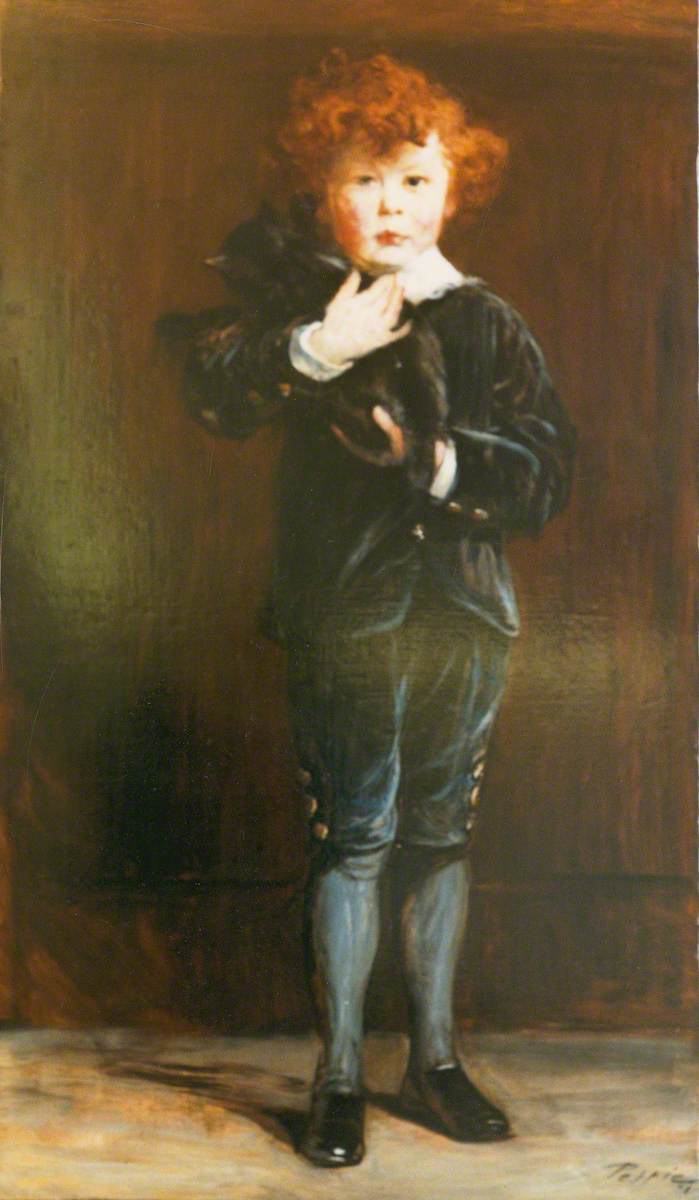The painting depicts a young boy of Caucasian descent with curly, red hair standing on a grayish floor with hints of green and orange. He is holding a black cat against his right shoulder, with the cat's head resting over his shoulder. The boy is dressed in 18th or 19th-century attire; he wears knee-length dark blue breeches with three orange buttons on each side, light blue knee-high socks or tights, and shiny black dress shoes. His upper body is clad in a dark blue velvet jacket adorned with numerous orange-gold buttons, over a white shirt featuring a high, lace collar. The background consists of a wall painted in shades of reddish-brown, giving it a wooden appearance. The child's pale skin catches light from the right side of the canvas, and his gaze is directed slightly off to the left. The bottom right corner of the painting features an illegible artist's signature, suggesting the image is of museum quality.